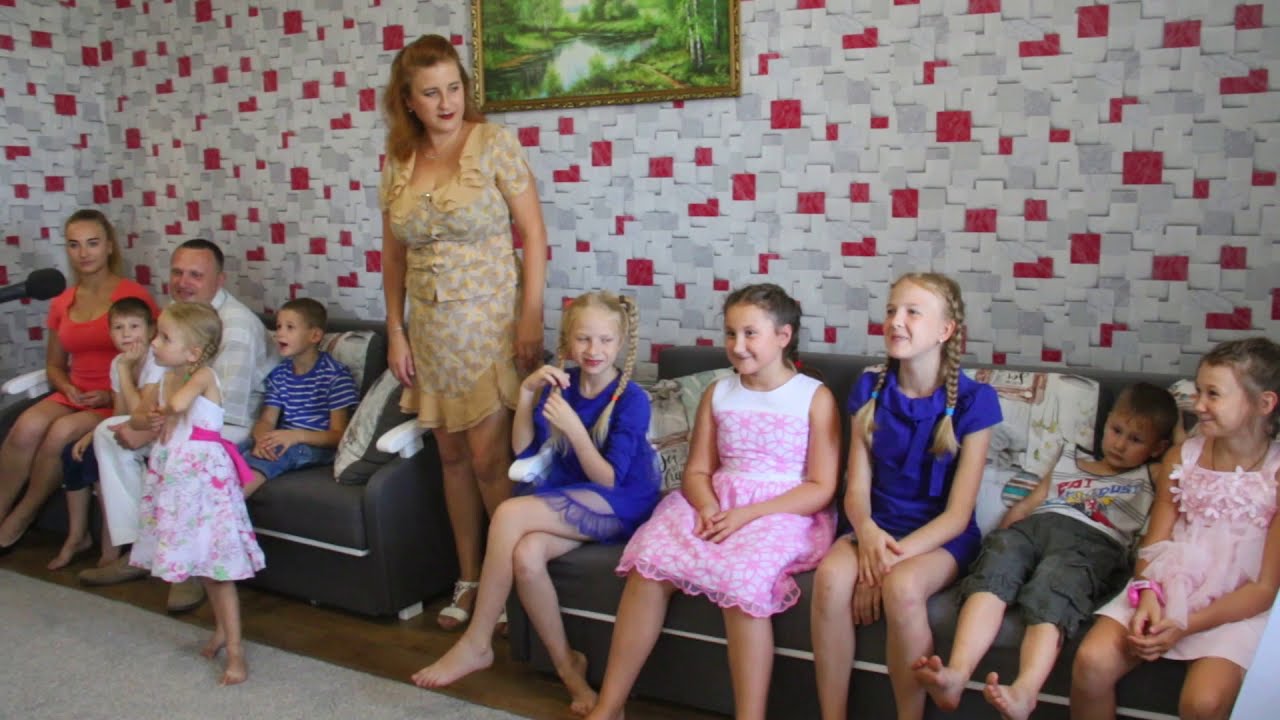In this image, two dark couches are positioned with a small space between them. The couch on the right is crowded with several kids, predominantly girls dressed in blue or pink dresses, and a solitary boy who seems somewhat out of place. On the left couch, there is the appearance of a family setting: three kids, two adults - a woman in a red dress and a man in a white shirt - with another child nestled between them. Standing in front of the left couch, a young girl in a pink dress looks upward, seemingly at a microphone emerging from the left side of the frame. Between the two couches stands a woman in a gold or tan dress with white shoes. Her gaze is directed at the kids on the right couch. Behind her, the wall features a distinct pattern of red, white, and gray squares, akin to post-it notes, alongside a nature scene encased in a gold frame.